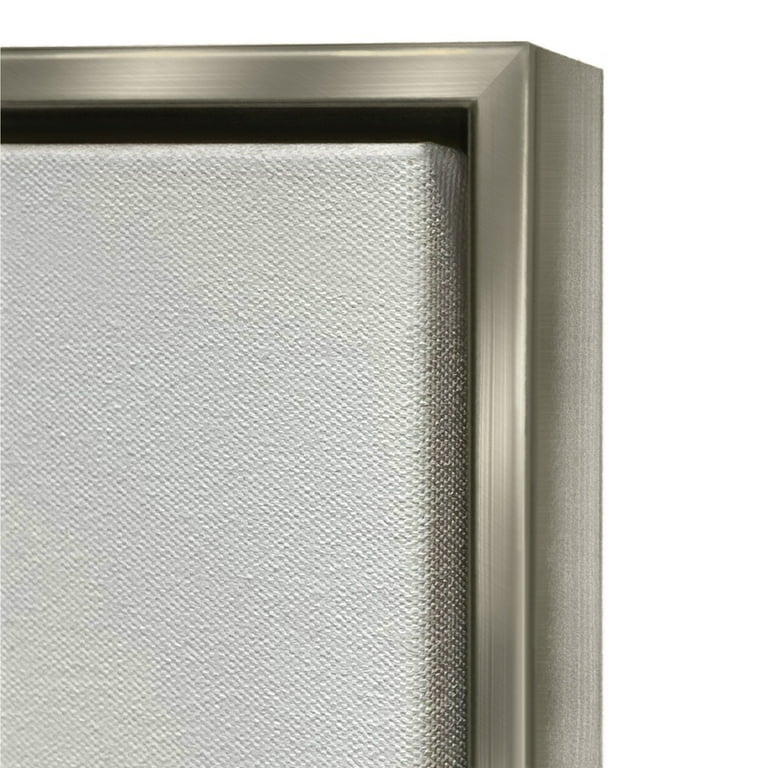The image showcases a partially visible geometric object, prominently featuring what looks like a framed panel with a cushioned insert, or possibly the front of a speaker. The frame is angular, right-angled, and metallic-looking, with a glossy gray finish, though it could be wood painted gray. The panel itself is rectangular, with a coarse-textured, spongy-looking white material inside, reminiscent of a speaker cover. There is a noticeable black gap at the top between the gray frame and the white insert, and smaller gaps on the sides. The product is placed towards the left side of the image, with the frame's corner positioned at the upper right of the photo. The photo’s aesthetic is monochromatic, playing with shades of black, white, and gray, set against a plain white background.